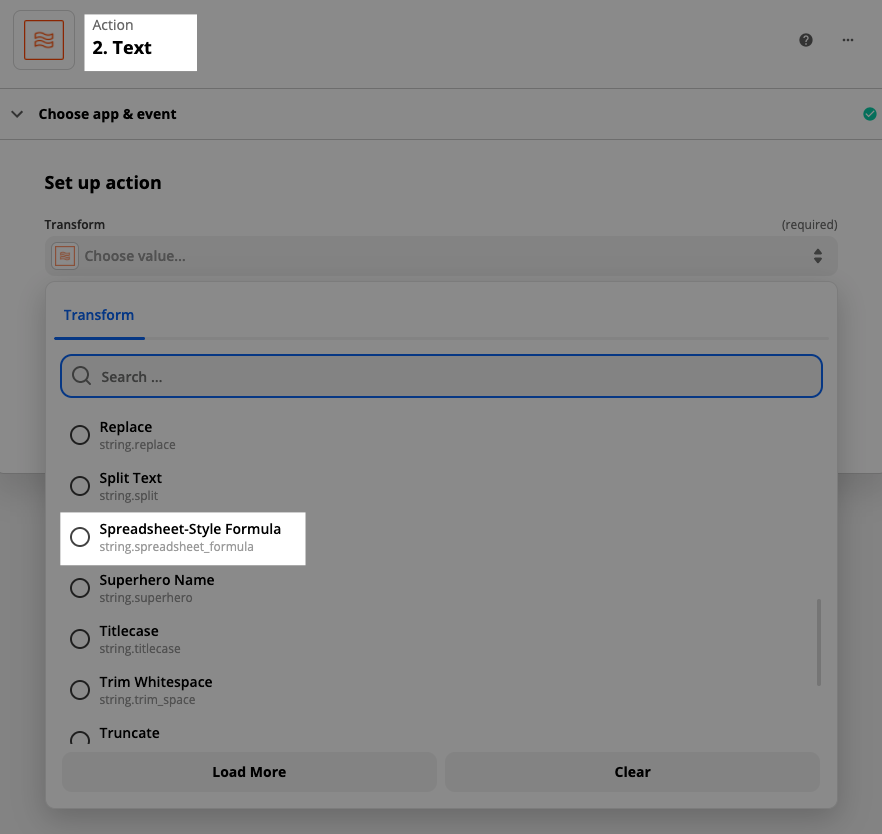The image features a predominantly shadow gray background with various elements and text that appear to be part of a user interface, possibly for a software application. In the upper left corner, there is a small orange square containing horizontal lines, adjacent to a white box with the word "Action" beside it. Below this, bold text displays the number "2" followed by the word "Text". 

Continuing downward, black text reads "Choose app and event," and beneath this line, it states "Set up action." The word "Transform" is listed next, followed by another orange box that includes "Choose value..." with the word "Required" in parentheses. The word "Transform" appears again, this time underlined and in blue. Accompanying this is a notably long search bar.

Further down, a circle icon is next to the word "Replace" with "String Replace" written underneath. Another circle is beside the text "Split Text." Highlighted in white, a small circle precedes the phrase "Spreadsheet style formula," followed by options such as "Superhero name," "Title case," "Trim white space," and "TRUNCATE" with a misspelling. 

The final interactive options include "Load more" to the left and "Clear" inside a box to the right.